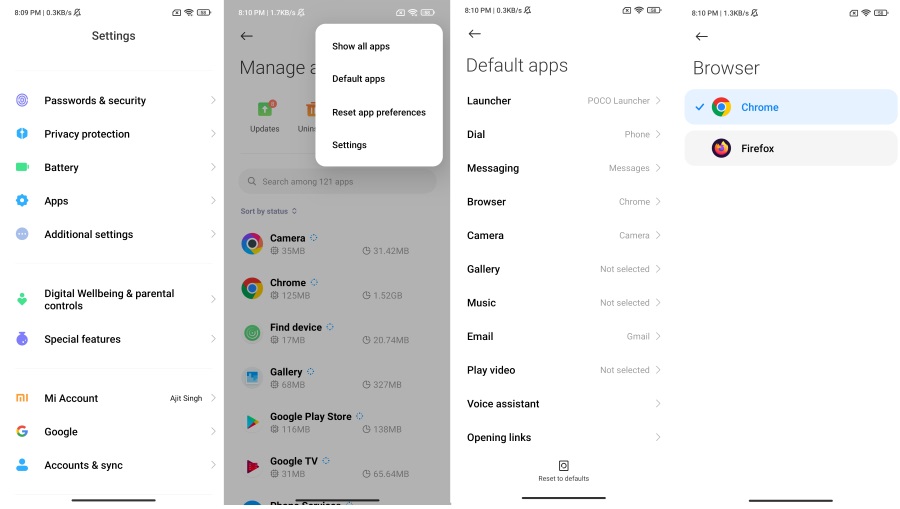A detailed caption of the image could be:

"This collage showcases a collection of cell phone settings panel screenshots. On the far left, a narrow screenshot displays the main 'Settings' menu on a white background. The options listed vertically include: 'Passwords and Security,' 'Privacy Protection,' 'Battery,' 'Apps,' 'Additional Settings,' 'Digital Wellbeing and Parental Controls,' 'Special Features,' 'Mi Account,' 'Google,' and 'Accounts & Sync.'

The second screenshot from the left is overlaid with a gray filter and features a dropdown menu in the top-right corner. This menu offers options like 'Show All Apps,' 'Default Apps,' 'Reset App Preferences,' and 'Settings.' Positioned behind this menu, the screen reveals the 'Manage All Apps' tab within the settings.

To its right, the third screenshot highlights the 'Default Apps' section, listing the default applications selected for various functions.

The fourth and final screenshot, located on the far right, focuses specifically on the 'Browser' settings. It indicates that the default browser is set to Chrome, with Firefox listed as an alternative option below it."